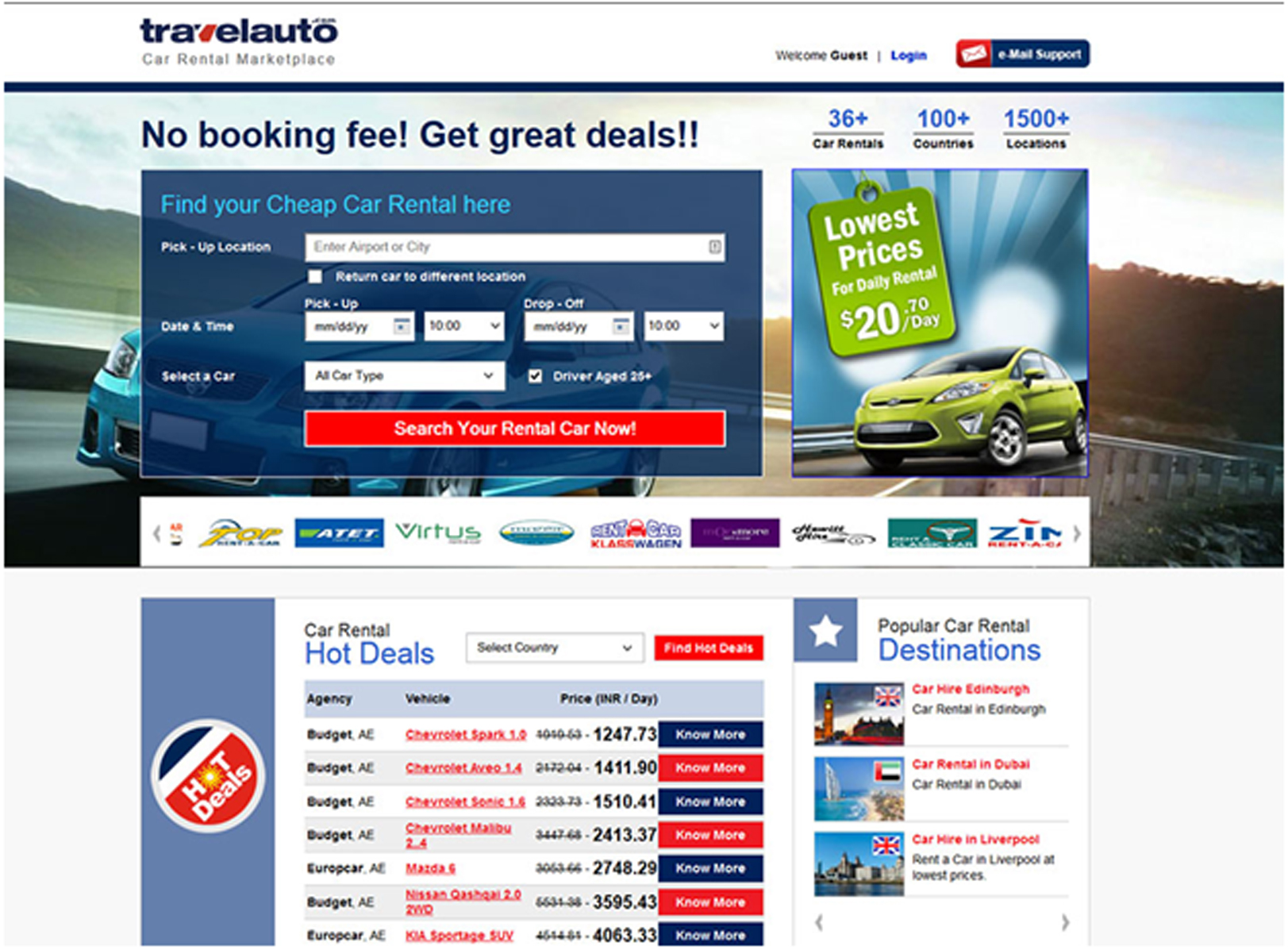**Travel Auto Car Rental Marketplace Web Page Overview:**

In this screenshot from the Travel Auto Car Rental Marketplace website, various elements are laid out to provide a comprehensive car rental booking experience. 

**Top Navigation:**
On the top-right corner, there are options for "Welcome Guest," a login button, and an email link for customer support. These elements appear as a pop-up overlaying a banner that spans the webpage.

**Banner Image:**
The banner features a blue economy car driving on a freeway in daylight, emphasizing the dynamic and adventurous spirit of car rentals.

**Pop-Up Information:**
Overlaying the banner is a noticeable pop-up with promotional messages:
- "No booking fee! Get great deals!!"
- "Find your cheap car rental here."

**Booking Form:**
Below the promotional pop-up, there is a detailed booking form which includes:
- A "Pick-up Location" box.
- An option to check "Return car to different location."
- Date and time selectors for both pick-up and drop-off, with respective dropdown boxes for the month, date, and year.
- "Select the car type" dropdown menu.
- A checkbox labeled "Driver age 20+."
- A prominent red button stating "Search your rental car now!"

**Additional Information:**
To the right of the booking form, there is a summary showcasing the availability and prices:
- "36+ car rentals in 100+ countries, 1,500+ locations."
- A green tag highlighting the "Lowest Price Daily Rental," starting at $20.70 per day along with an image of a vehicle.

**Advertisements:**
Several ads are displayed below, including:
- Companies like ATET and Virtus, along with a few others not clearly visible.

**Hot Deals:**
A "Car Rental Hot Deals" section presents selectable options:
- A dropdown menu to "Select Country."
- A red button prompting "Find Hot Deals."
- Listings categorized under "Agency," "Vehicle," and "Price," with repetitive mentions of "Budget AC."

**Popular Destinations:**
To the right side, there's a section dedicated to "Popular Car Rental Destinations."

Overall, the web page is designed to facilitate easy navigation and quick booking for users, promoting both cost savings and convenience.